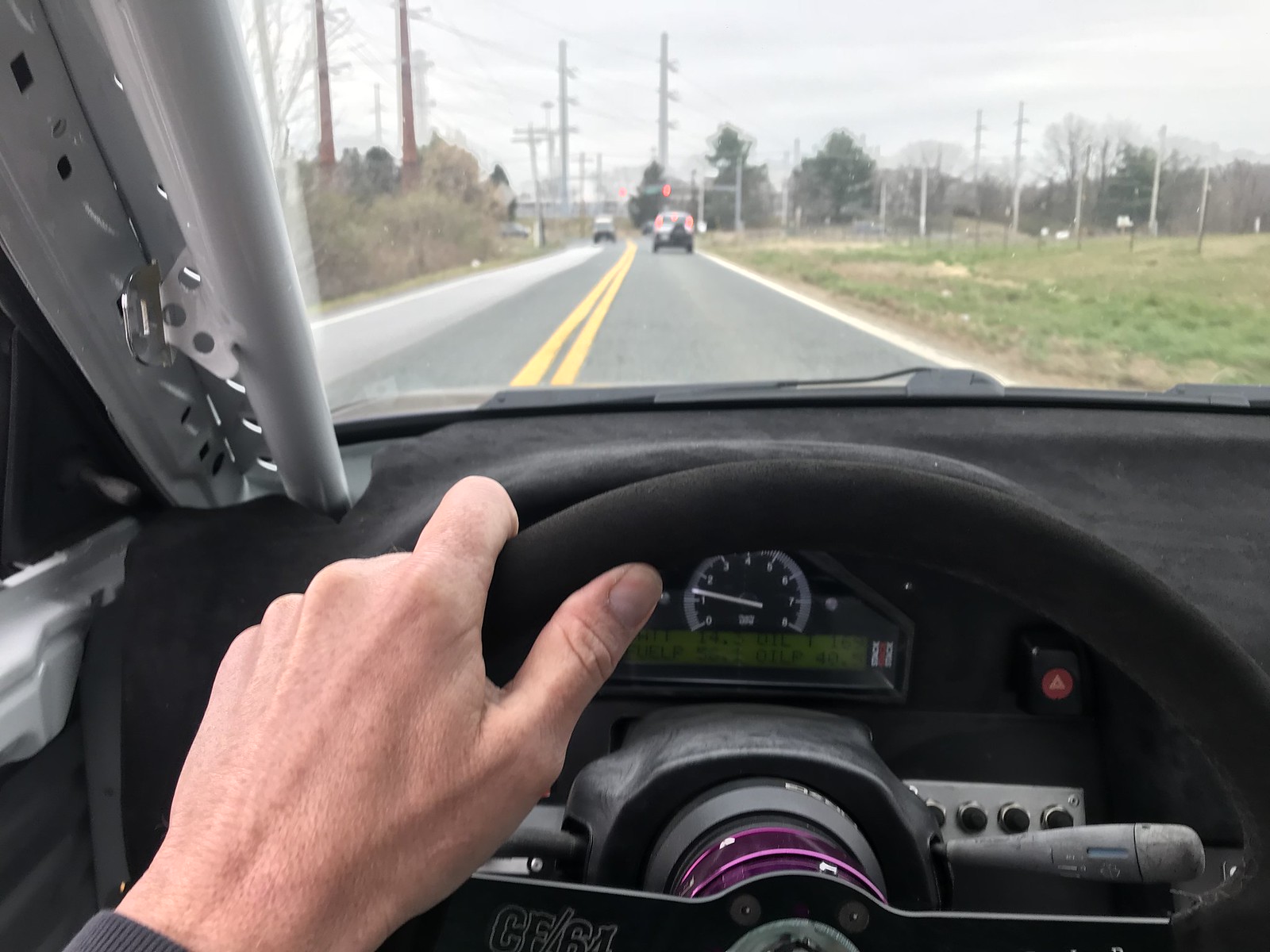This vivid color photograph captures a scene from the perspective of the driver in a sporty, custom-modified car traveling on a rural road. The driver's seat is situated on the left-hand side of the vehicle, which is driving on the right side of the road, visible through the windshield. The car’s sleek black steering wheel, held at the 10 o'clock position by a spotted hand, is prominently featured. The hand, possibly belonging to someone in their 30s or older, is surrounded by the robust, race car-like build of the vehicle's interior. 

Ahead, the road is marked with two solid yellow lines on the left, bordered by grass and some bushes, extending into a countryside setting devoid of fences. A set of traffic lights ahead glow red, signaling the driver to stop. A car is seen ahead, waiting at the intersection, with telephone lines and a stop sign further detailing the rural scene. The vehicle's dashboard, featuring black and silver details with an analog speedometer marked from 0 to 8, includes a small green screen displaying partial texts like "OILP 40." The dashboard also has black and purple accents, along with a red triangle button, contributing to the sporty aesthetic of the car. This detailed capture vividly portrays the experience and environment of the driver from a first-person perspective.